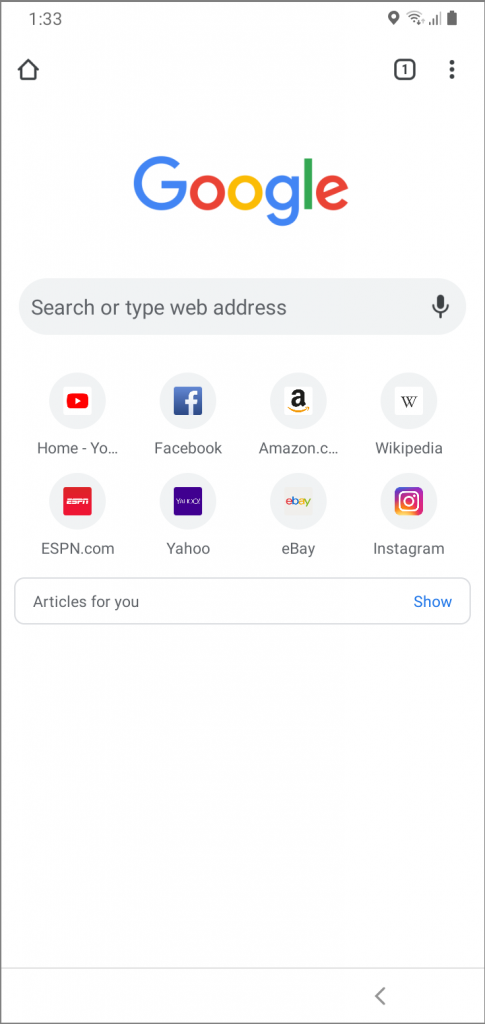A screenshot from a smartphone reveals the Google search homepage, characterized by the standard smartphone status icons at the top, including the time, battery level, and network strength. Dominating the screen is the familiar Google logo above the central search bar where users can input queries or web addresses. Below the search bar, shortcut icons for the user's most visited sites are displayed, including YouTube, Facebook, Amazon, Wikipedia, ESPN, Yahoo, eBay, and Instagram, enabling direct navigation. An "Articles for you" section is visible but collapsed, indicated by a blue "Show" button that, when tapped, would display personalized content. The clean, white background suggests no special Google doodle is featured on this day. Additionally, a home icon situated in the top left corner offers a quick return to the user's designated homepage.